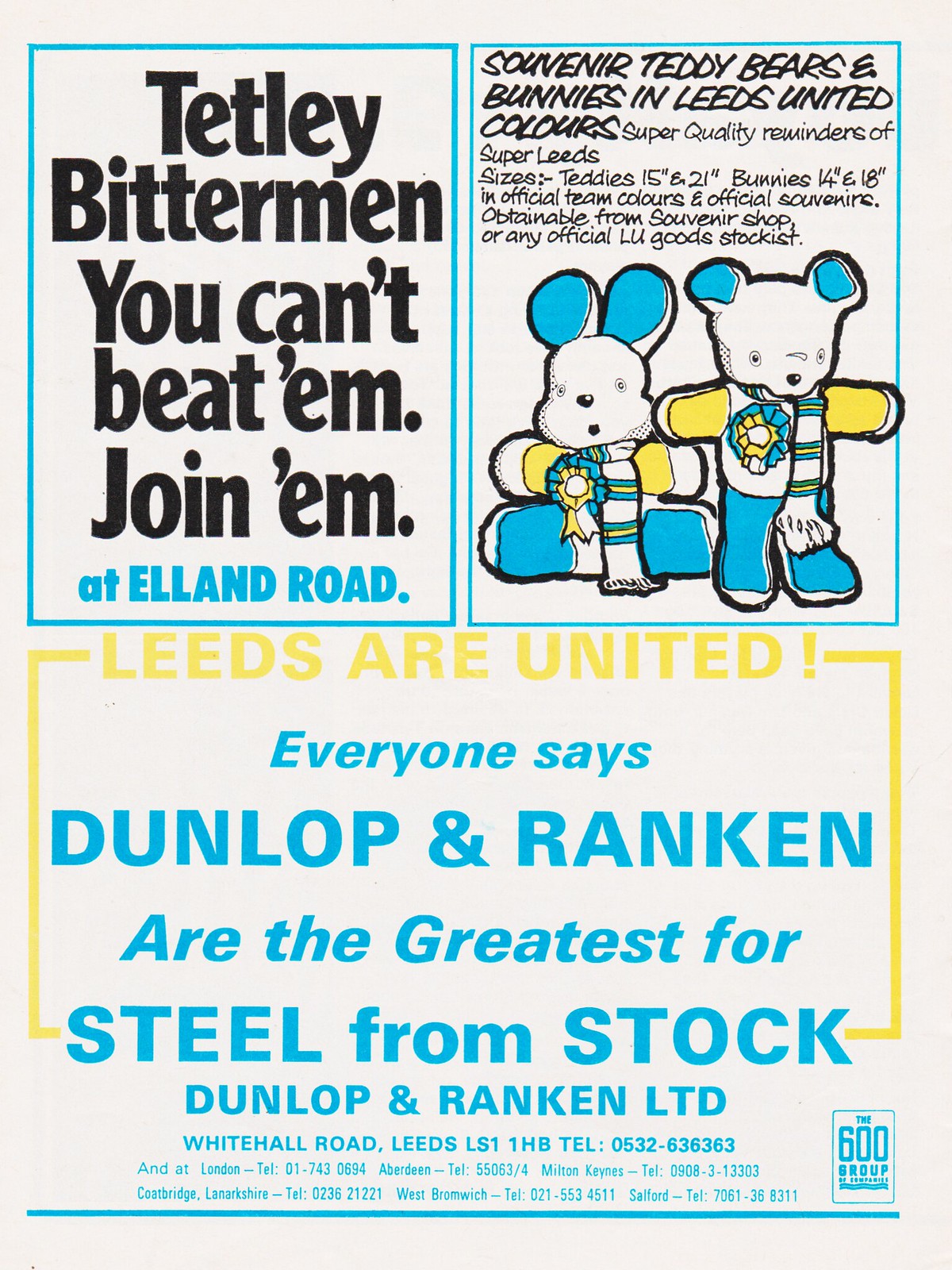The image appears to be a magazine advertisement divided into three sections. The top half of the page is split into two segments. In the top left segment, there is a blue-bordered square frame with the text "Tetley Bitterman, You Can't Beat Him, Join Him" printed. Below this, it reads "at Elland Road" in blue text. The top right segment features another light blue-bordered square frame, with black text advertising "Souvenir Teddy Bears and Bunnies in Leeds United Colors." This text promotes "Super Quality Reminders of Super Leeds" and mentions sizes for the teddies (15 and 21 inches) and bunnies (14 and 18 inches). These items are available in official team colors and can be purchased from a souvenir shop or any official Loo Goods stock list.

In the bottom half of the image, it says, "Leeds are United." The text continues with "Everyone says Dunlop and Rankin are the greatest for steel from stock. Dunlop and Rankin Limited, White Hall Road, Leeds, LS1 1HB," followed by a telephone number. The advertisement uses colors blue, yellow, and black, and features images of the teddy bears and bunnies in Leeds United colors.